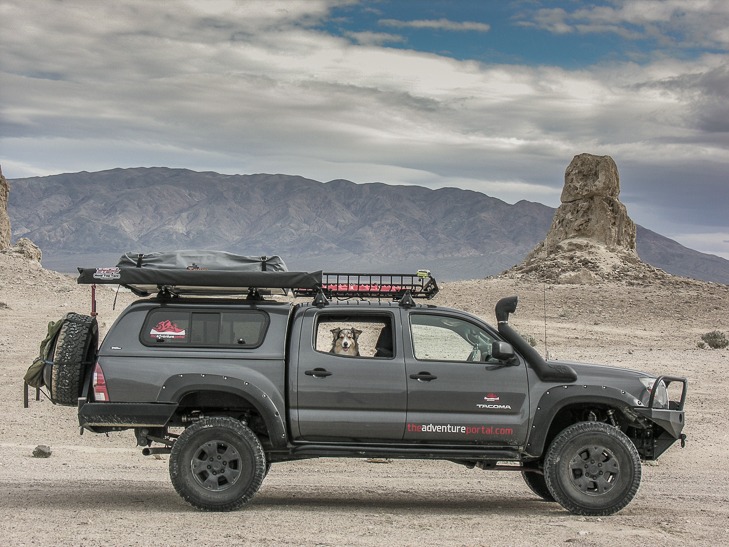The image captures a detailed scene set in a desolate, desert landscape during the daytime. The sky is predominantly gray and overcast with just a hint of dark blue peeking through the clouds. A rugged mountain range forms the backdrop, its arid and gray appearance emphasized by the starkness of the rocky terrain below.

In the foreground, a dark gray Toyota Tacoma pickup truck is parked, its orientation showing the front end angling to the right and the rear to the left. The truck is equipped with various accessories: a spare tire mounted on the back, a bike rack on top, and luggage racks. Notably, there is text on the vehicle, prominently displayed on the front passenger-side door, reading "theadventureportal.com."

The truck’s windows are rolled down, revealing an Australian Shepherd dog sitting in the back seat, gazing out attentively. This adds a touch of life and companionship to the otherwise remote and still setting. The scene suggests an adventurous outing, possibly an event, with the truck poised for exploration amid the natural stone formations and sandy terrain.